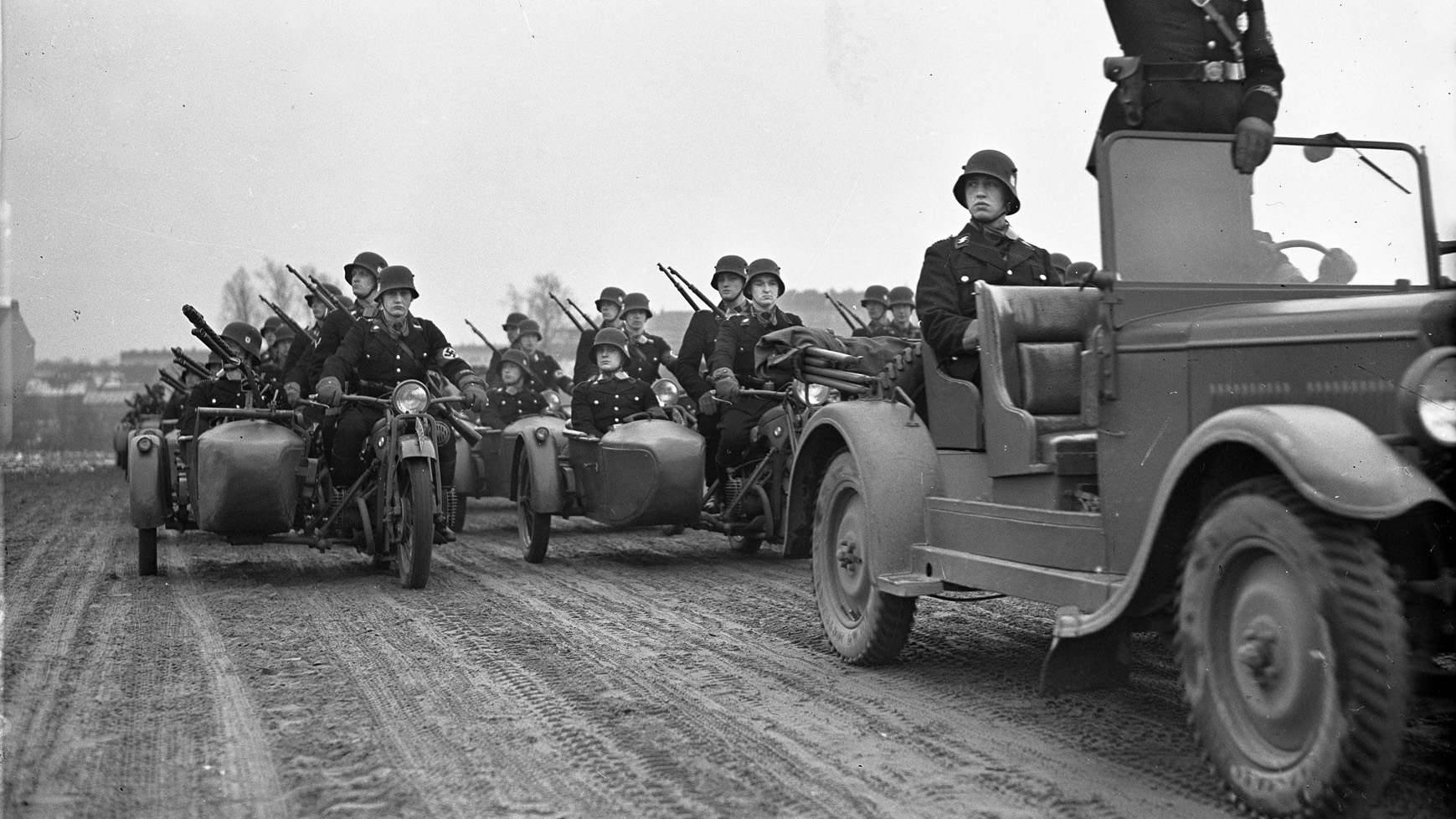This black-and-white photograph, likely from the 1940s or 1950s, captures a somber and regimented military procession moving along a wide, well-traveled dirt road. In the foreground, a Jeep, possibly a Willys, is prominently featured with a uniformed officer standing up next to the driver, and another officer seated in the back. All soldiers are clad in dark military uniforms with rounded helmets. Trailing behind the Jeep is a motorcade of military motorcycles with sidecars, forming three or four orderly rows that extend into the background. The image exudes a dark and ominous atmosphere as the soldiers, poised and ready, seem to be heading off to war.